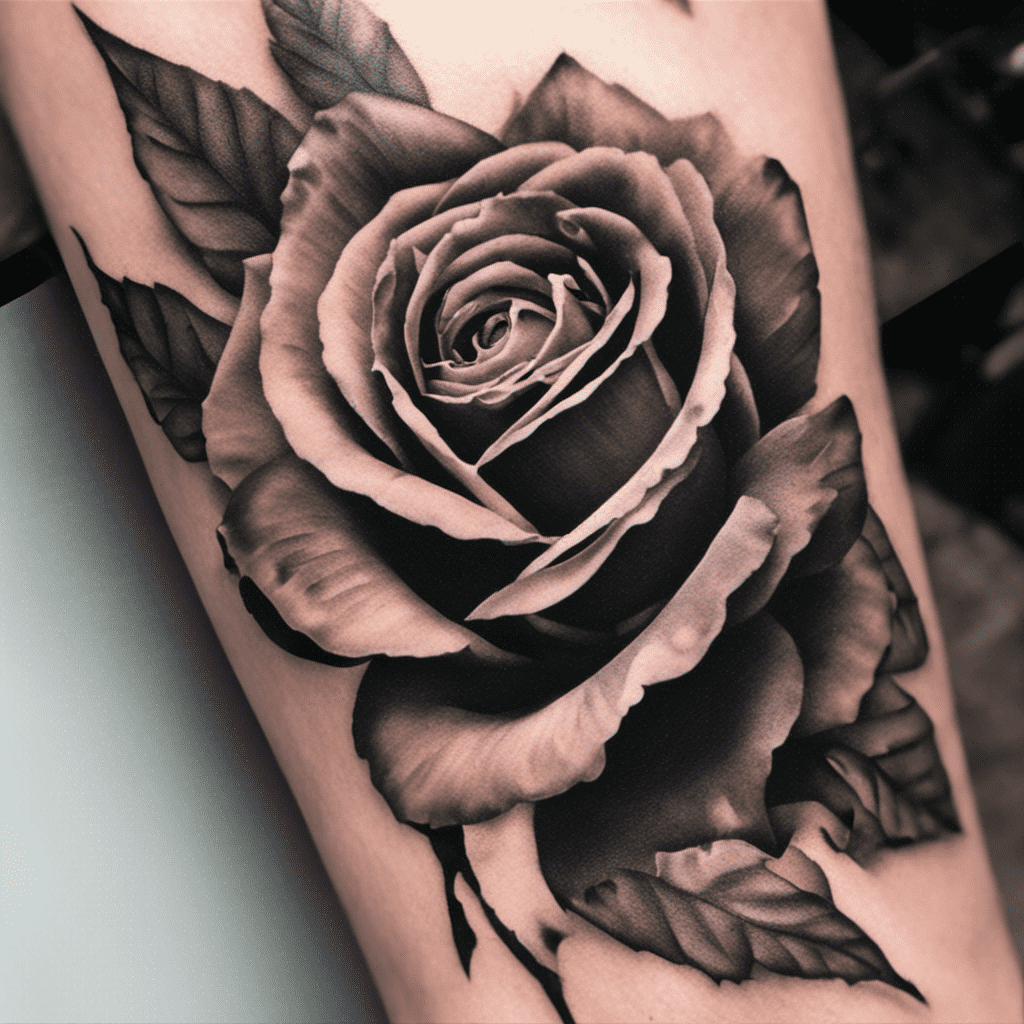This image shows a close-up of an intricate black and gray rose tattoo on a Caucasian individual's arm, possibly the forearm or even the top half of the hand. The large rose occupies most of the visible area, featuring tightly wound petals at the center that gradually unfurl outward, showcasing exquisite shading in gray and white ink. The design includes a few leaves and stem details both above and below the rose, enhancing its natural appearance. The arm rests on a turquoise blue stand in the image, emphasizing the stark contrast of the tattoo against the skin. There also seems to be an imaginative addition where ink appears to be dripping from the bottom left petal of the rose, adding an element of dynamic artistry to the piece.